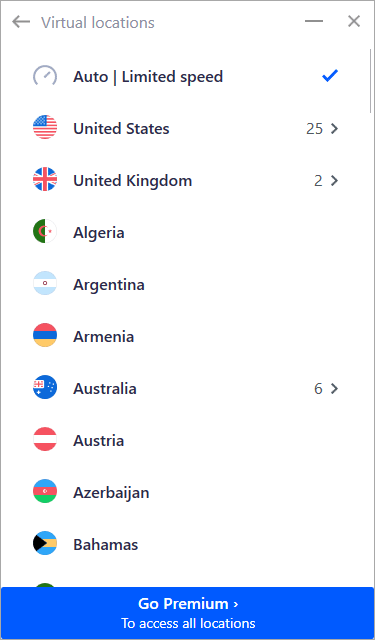Screenshot of a Category from a Website Listing Virtual Locations:

At the very top of the image, the heading "Virtual Locations" is prominently displayed. The interface includes navigational elements such as a back arrow on the left and an X on the right, allowing users to return to the previous screen or close the current window. Below the heading, there is a blue check mark indicating a selected option labeled "Auto and limited speed."

The list of virtual locations appears beneath this option, each accompanied by their respective national flags. Notable entries include:
- United States, with the number 25 next to it
- United Kingdom, with the number 2
- Australia, with the number 6

Several countries are also listed without numbers next to their names, indicating no available connection or server count:
- Algeria
- Argentina
- Armenia
- Austria
- Azerbaijan
- Bahamas (partially obscured by another element of the interface)

A prominent blue bar covers part of the list, containing a "Go Premium" button. Text on the bar reads, "To access all locations,” accompanied by an arrow icon, suggesting that further actions or premium subscription is required to unlock additional virtual locations.